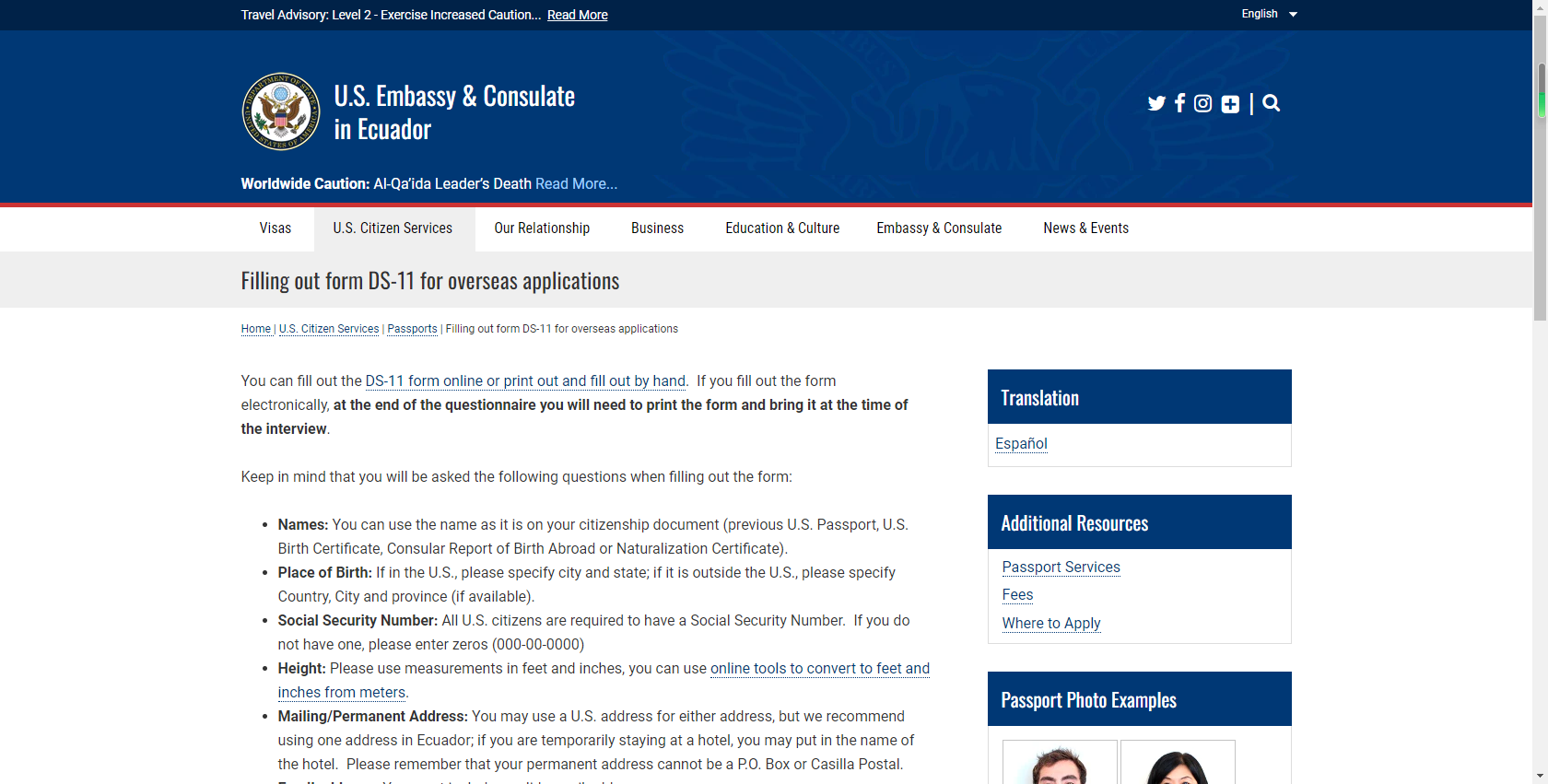The image depicts the homepage of the U.S. Embassy and Consulate in Ecuador's website. The top section of the site features several navigational headings including "Visa," "U.S. Citizen Services," "Our Relationship," "Business," "Education and Culture," "Embassy and Consulate," and "News and Events." Social media icons located in the top right corner provide links to the Embassy's Twitter, Facebook, and Instagram pages, along with a search button to facilitate easy navigation.

Dominating the main section of the screen is detailed information about completing the DS-11 form for overseas applications. The "U.S. Citizen Services" tab is highlighted, indicating the current section selected. The content comprises a paragraph of instructional text and some emphasized phrases in bold for clarity. Instructions such as "At the end of the questionnaire, you will need to print the form and bring it at the time of the interview" stand out in bold text. Additionally, the form-filling process includes personal details like names, places of birth, social security numbers, and height.